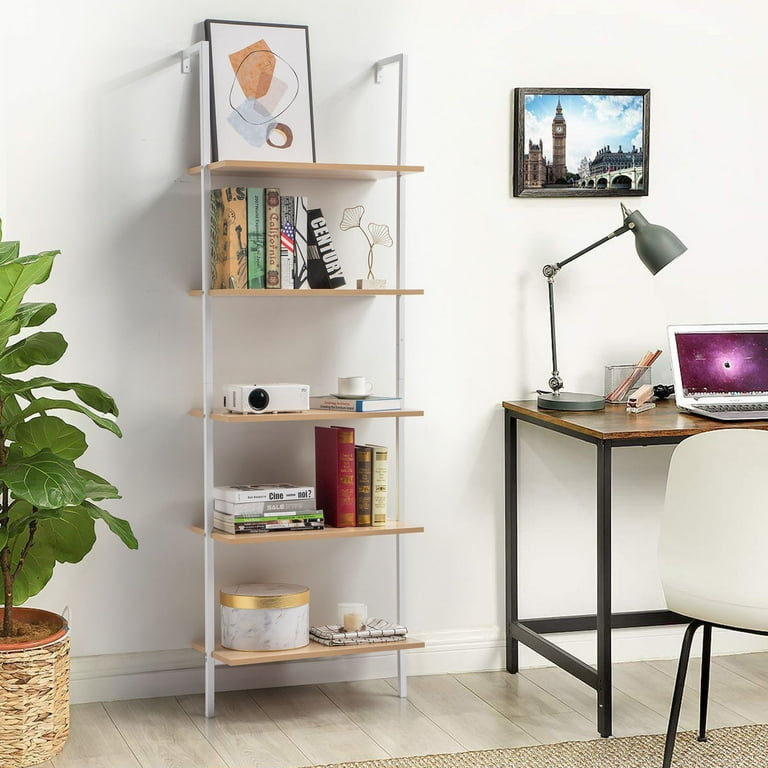This square photograph, measuring approximately 5 to 6 inches on each side, captures an indoor room that appears to be used as an office or den. The setting features a light grayish-brown wooden floor, complemented by an eggshell white wall that serves as the backdrop. In the bottom right-hand corner of the image, a small section of a brown rug is visible.

On the left side of the room stands a large potted plant with expansive, green waxy leaves, housed in a wicker basket. Adjacent to the plant is a vertical bookshelf attached to the wall. The bookshelf consists of multiple wooden shelves supported by a black metal rack. At the top sits a framed picture, while the remaining shelves display an assortment of books, trinkets, and what appears to be a white projector. The bottom shelf holds a cylindrical box with a white marble side and a gold top.

To the right of the bookshelf is a black metal desk featuring a brown wooden top. On this desk, a gray desk lamp, a laptop, and various office supplies including a pink stapler can be seen. A white chair with black legs sits in front of the desk, resting on a beige rug. Above the desk hangs a horizontally-oriented framed picture of Big Ben in London.

The detailed elements and organized arrangement create a cozy and functional workspace within the room.